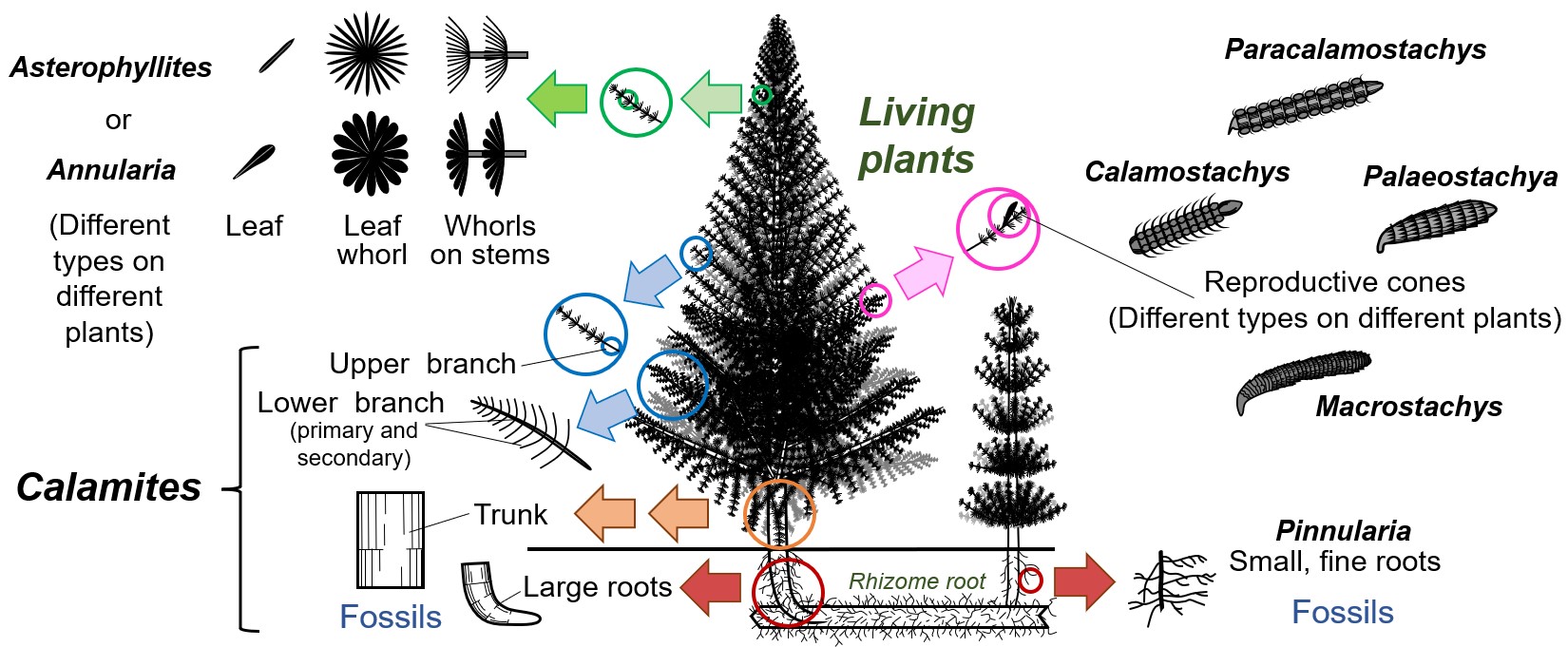The image is a detailed, colorful digital illustration of living plants, prominently featuring a central tree-like plant. It serves as an educational poster, meticulously labeling various parts of the plant and tree anatomy with arrows and text, making it somewhat confusing for those unfamiliar. The illustration includes sections on different types of plants, like astrophytes and annularia, and names specific plant parts such as the leaf, leaf whorls on stems, and reproductive cones. Noteworthy scientific terms appear, like calomastica and pericalomastasia for the cones, and pinulera for small fine roots. The diagram spans from the large roots and trunk at the bottom, through the middle section of the plant, to the upper branches, with additional notes on the leaves and flowers. It captures an intricate portrayal of plant biology, resembling a pine tree with various cones depicted on the right and left sides.